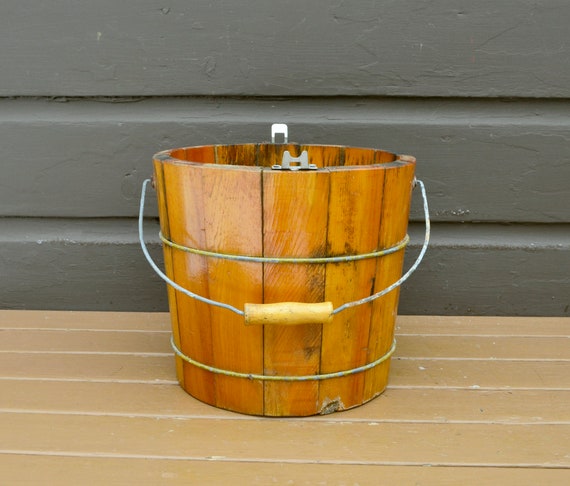A utilitarian scene is set against a gray wall, dominated by an old-fashioned wooden ice cream maker. This rustic device, meticulously crafted from vertical slats of brown wood, boasts a robust design secured by two horizontal metal bands. A conspicuous feature is its substantial metal handle and a central wooden crank, hinting at its function. A close inspection reveals a chipped section at the bottom, whispering tales of its storied past. The interior, visible just slightly, is lined with gray material and features a small latch mechanism. Resting nearby is a light brown bench, completing this nostalgic tableau.